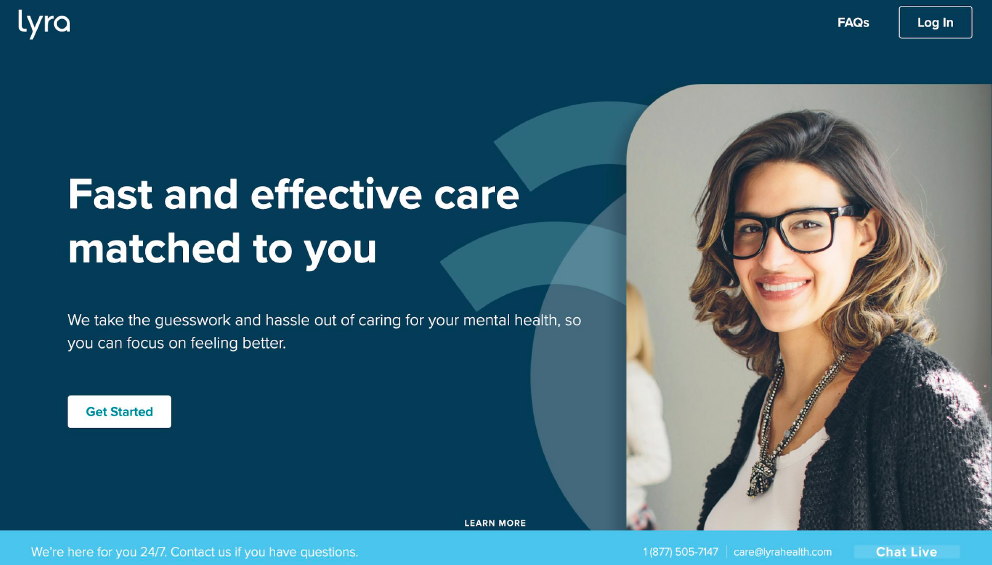Here is a polished and detailed descriptive caption for the image:

---

This is a screenshot of a landing page for a website called Lyra (L-Y-R-A). In the upper left-hand corner, there is a text logo. In the upper right-hand corner, there are links for FAQs and a rectangular login button with white text outlined by a thin white border. The background of the page is a dark blue, and at the very bottom, there is a light blue footer. The footer states, "We're here for you 24/7. Contact us if you have questions," and includes a phone number (1-887-505-7147), an email address (care@lyrahealth.com), and a button for live chat.

The main visual features a photograph of a woman who is smiling. She has wavy, shoulder-length hair and is wearing dark black, plastic-rimmed glasses. She is dressed in a fluffy dark gray cashmere sweater, with a beaded necklace that has a knot in the center, and a scoop neck top or possibly a white tank top underneath. Her body is facing towards the left. In the background, there is another woman, partially cut off, who has her face turned towards the camera, smiling broadly. She appears to be around 35 years old.

To the left of the image, there is large text that reads, "Fast and effective care matched to you." Below this, in smaller text, it says, "We take the guesswork and hassle out of caring for your mental health so you can focus on feeling better." There is also a "Get Started" button, featuring white and blue text. Behind the photograph are two curved arcs and a circle design, adding a visual element to the composition.

---